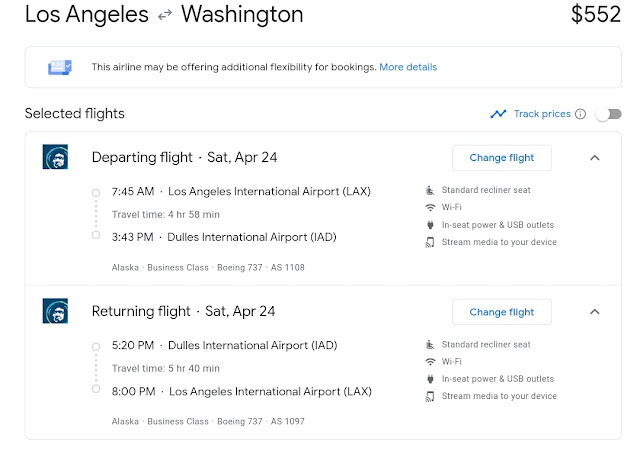The image features a detailed round-trip flight itinerary from Los Angeles (LAX) to Washington, D.C. (Dulles International Airport - IAD) priced at $552. It has a clean, white background with a box below stating that the airline may offer additional flexibility for bookings. On the right, there's an option to "Track Prices," although the button is not activated.

**Outbound Flight:**
- **Date:** Saturday, April 24th
- **Departure:** 7:45 AM (LAX)
- **Duration:** 4 hours and 58 minutes
- **Arrival:** 3:43 PM (IAD)
- **Aircraft:** Boeing 737
- **Amenities:** Standard recliner seat, Wi-Fi, in-seat power and USB outlets, streaming media to your device

**Return Flight:**
- **Date:** Same day, April 24th
- **Departure:** 5:20 PM (IAD)
- **Duration:** 5 hours and 40 minutes
- **Arrival:** 8:00 PM (LAX)

Overall, the entire round-trip journey spans approximately 12 hours, allowing you to travel from Los Angeles to Washington, D.C. and back in a single day.